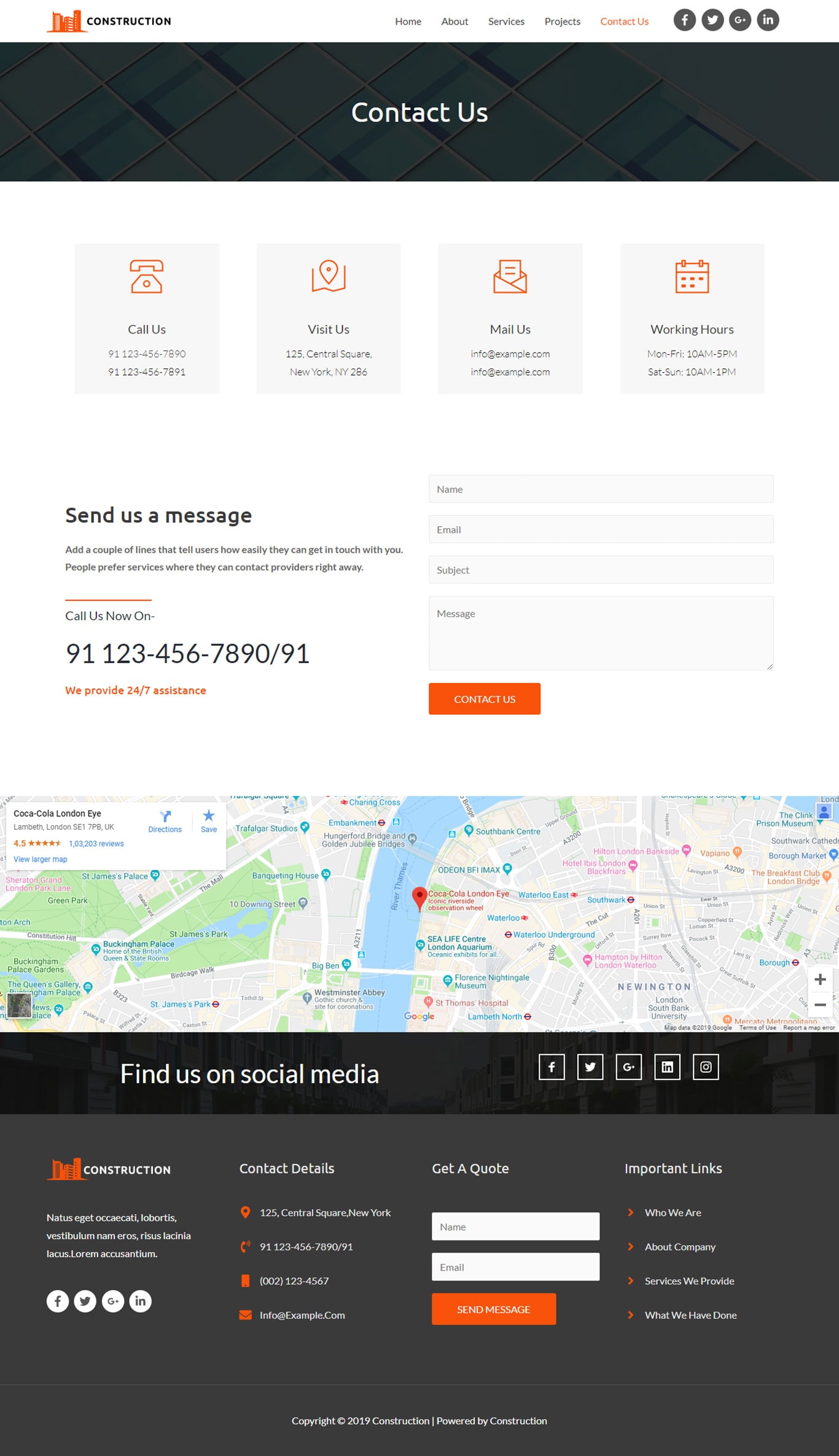The image features a header with a prominent black box at the top displaying the text "Contact Us." Next to this header is text that appears partially blurred but seems to mention "Construction Home" and a few other unclear elements. To the right of this text are social media icons, clearly identifiable as Facebook, Twitter, and LinkedIn, along with one unidentified icon. 

Below the header, there is a gray box containing an orange telephone icon followed by some text, and another gray box with a location icon and additional text. Further down, there are two more gray boxes with unspecified icons that are too blurry to identify, each accompanied by text.

To the left of these elements, the words "Send Us a Message" are displayed prominently along with a phone number: 31123-456-7890-91. Below this section, a map with a red location pin is shown, indicating a spot in the middle of a river. Beneath the map, there are several navigation links labeled "Find Us on Social Media," "Contact Detail," "Get a Quote," and "Important Links."